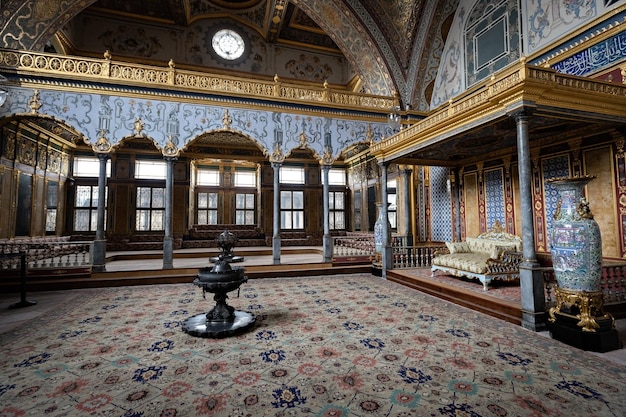The photograph captures the interior of a large, ornate building, possibly a place of worship such as a mosque, synagogue, or temple, distinguished by its lavish architectural details and elaborate decor. Central to the image is a black fountain or a similar ornamental structure positioned on an intricately designed Persian rug. The surrounding environment features light blue, blue, gray, gold, light brown, brown, red, and maroon hues.

On the right side of the image, there are two tall, intricately engraved blue pillars supporting a gold-accented overhang. Below the overhang sits an ornate gold couch. Adjacent to this area, two substantial gold and blue vases stand prominently, adding to the grandeur. The backdrop includes stained-glass circular windows near the top of the building’s towering domed ceilings, allowing natural daylight to fill the space. The left portion of the image reveals another gold balcony supported by intricately designed blue pillars, emphasizing the regal and opulent nature of this interior.